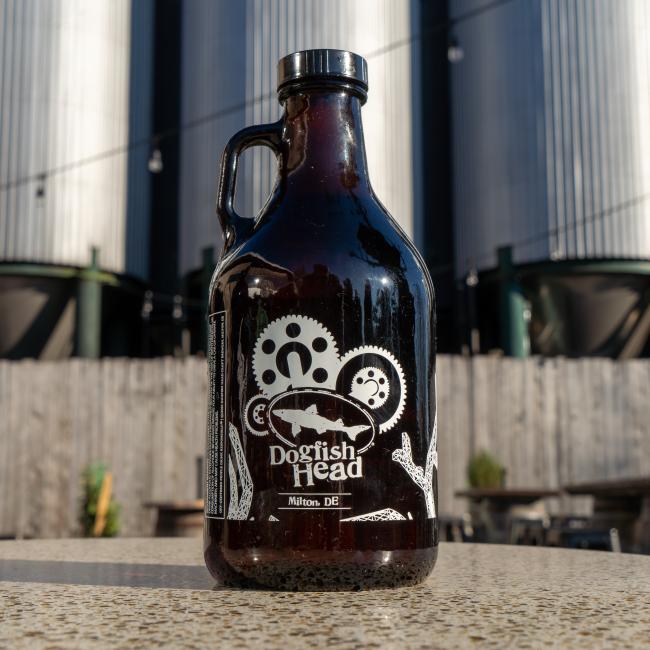This image showcases a dark brown glass growler of beer adorned with intricate white text and graphics. The growler features a handle near the bottleneck and has a black cap. The front of the growler prominently displays "Dogfish Head Milton, D.E." in white text, along with a computer-generated graphic of a shark encased in an oval. Surrounding the shark are several gears of varying sizes and pieces of coral on either side. Below the text, there's a small rock graphic on the bottom right side of the bottle. The bottle is placed on a granite tabletop in someone's backyard. The background reveals a fence and three large metallic brewing silos, with faintly visible machinery and a string of light bulbs attached to the fence. The photo captures the growler in sharp focus, while the outdoor elements appear slightly out of focus, giving context to the scene.